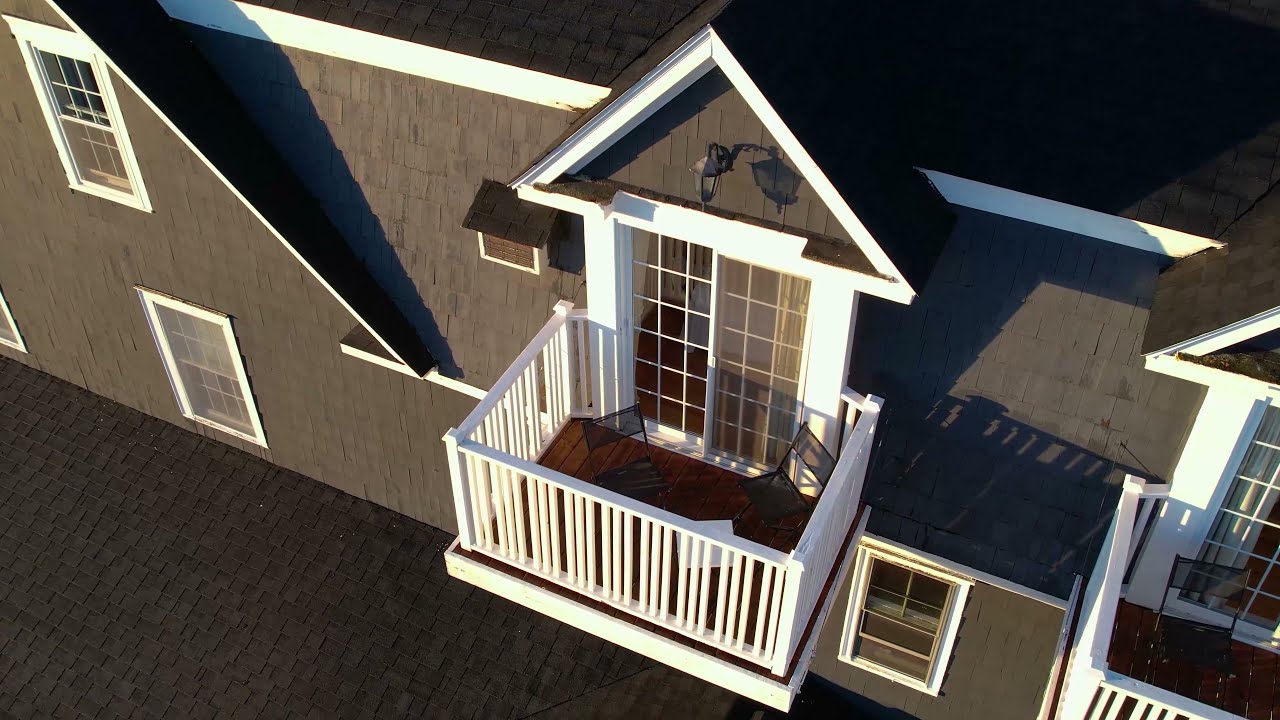This image, likely captured by a drone in the late evening, presents a detailed top-down view of a large, dark gray house with a pointy peak roof. The building extends diagonally from top-left to bottom-right, and is two stories tall, with a secondary balcony visible to the right. The sun, possibly positioned in the bottom-left or back-right, casts long shadows on the house, giving the dark gray exterior a lighter appearance. 

The main balcony, which features prominently in the image, is accented with white-walled sides and thin white rectangular bars arranged in a pattern of three, except at the corner edges where the pattern shifts to two bars. This balcony has a brown stained wooden floor and contains chairs, adding to the cozy ambiance. The balcony is accessed by two large, vertical rectangular windows, each divided into six sections by two thin vertical bars. Framing the windows is a white trim, which matches the overall white accents of the balcony.

Additionally, two lanterns are visible over the sliding door that leads to the balcony: one clearly seen in the center and another partially cropped by the image on the right. In contrast to the white features, the shingled parts of the roof, also visible in the lower-left corner, are dark gray, mirroring the primary façade of the house. The comprehensive view suggests that this substantial structure is likely a grand residence or a hotel, giving just a glimpse of its extensive architecture.